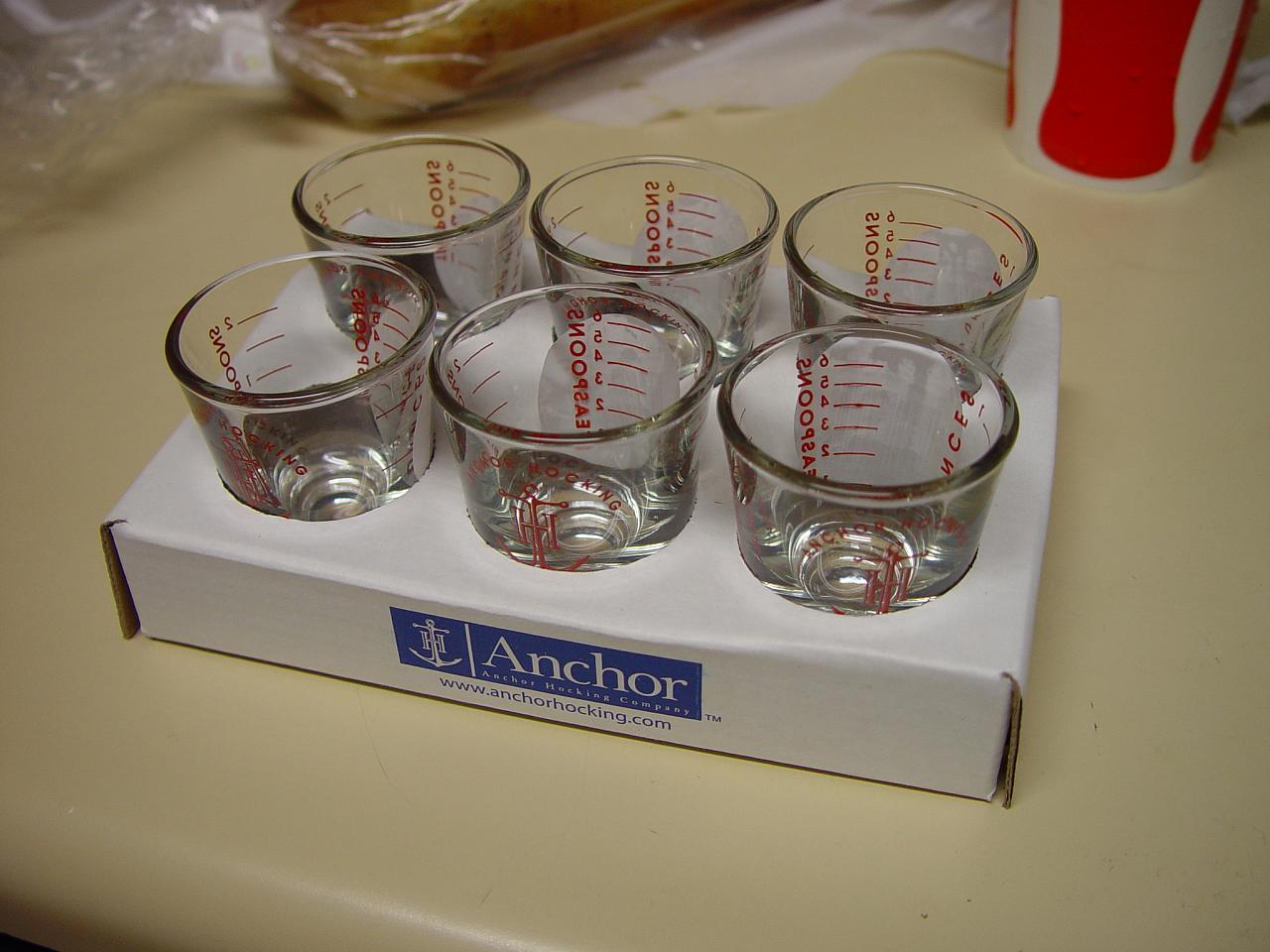The image depicts a set of six clear glass measuring cups with red measurement markings neatly arranged in a white cardboard tray. The tray displays a blue section on the front with the word "Anchor" written in white letters, accompanied by an illustration of an anchor, and the website "www.anchorhocking.com" below it. The measuring markings on the cups range from 6 to 2, descending vertically alongside red lines. The setup is on a cream-colored countertop. To the right of the tray, there's a partial view of a red and white paper cup, and to the left, there is a loaf of bread wrapped in clear plastic.